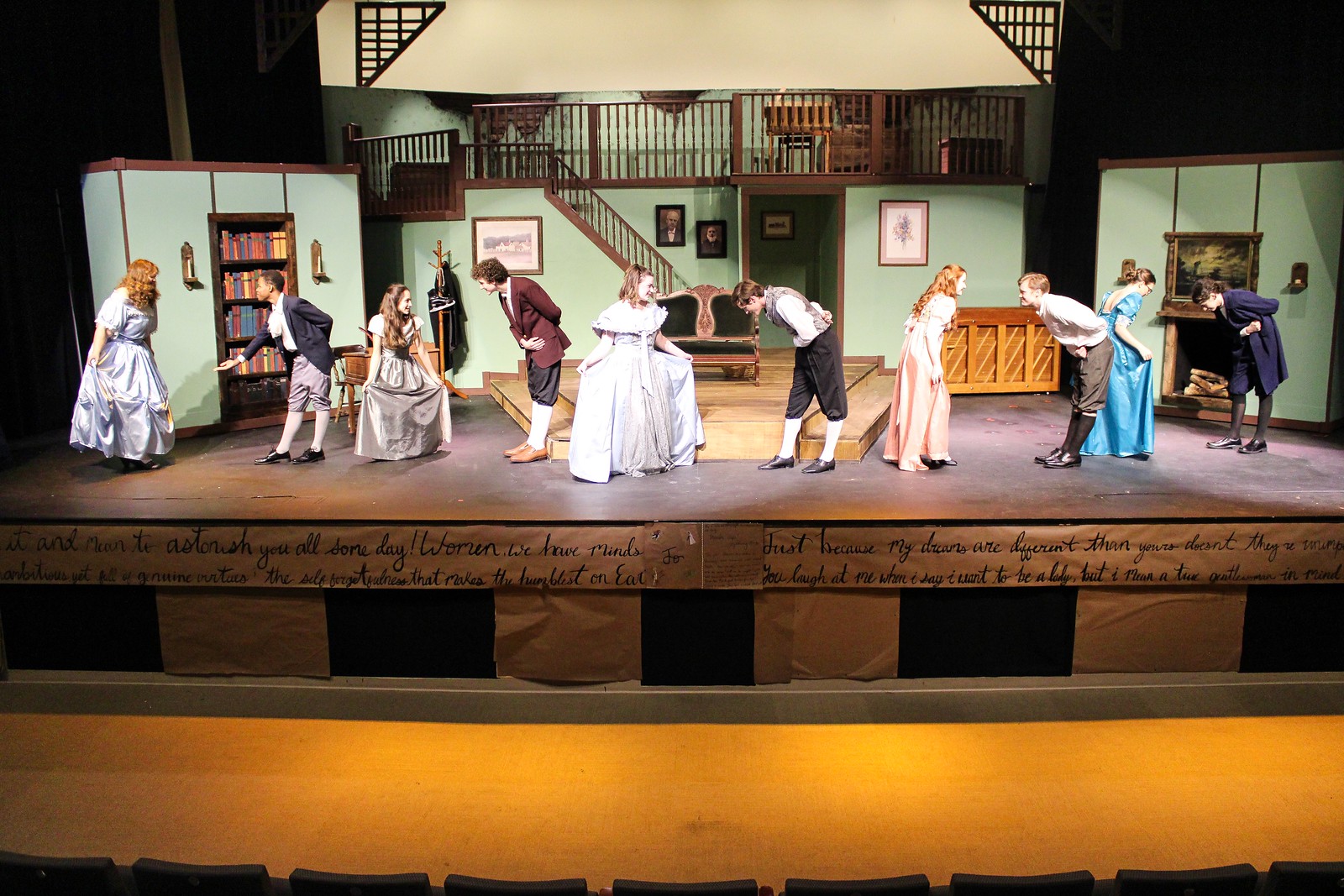This image depicts a scene from a theatrical performance set in the Victorian era. On the stage, which appears to be part of a high school performance judging by the actors' young ages, there are five couples arranged from left to right, each consisting of a man and a woman. The women are dressed in elaborate Victorian dresses, while the men sport pantaloons, ruffled shirts, suit jackets, and long stockings with shoes. The men are engaged in various courtly gestures—some are bowing, others extending their hands, and one is curtsying. The backdrop of the stage simulates an interior of a vintage home with green walls, wooden staircases leading to an open second floor, bookcases on the left, and a fireplace on the right. The stage itself has an old wooden floor and in front of it, there's a yellow area with paper inscribed with different words. The audience section can be seen but is unoccupied, suggesting the photo was taken during a rehearsal or before the performance commenced.